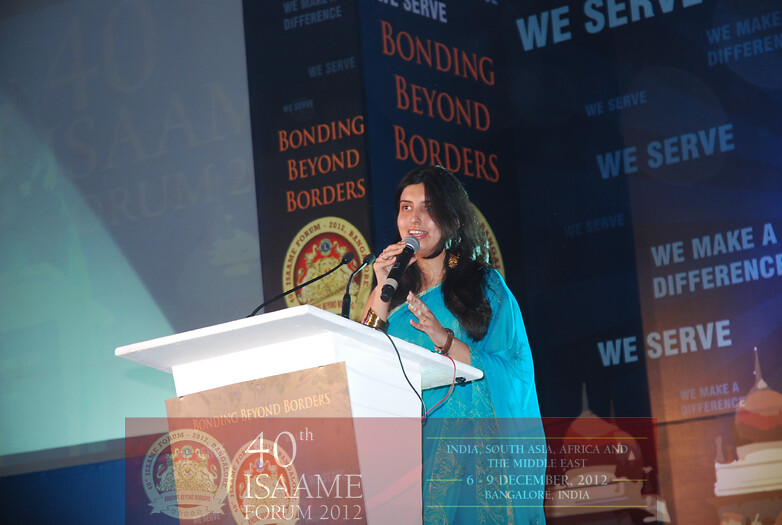In this color photograph taken in landscape orientation, a woman dressed in a turquoise-blue traditional sari gown with long dark hair stands at the center of the image. She is situated at a white podium, holding a microphone close to her lips and looking slightly upward to her left. The podium is equipped with two additional microphones. On her left, at the edge of the image, is a projector displaying the numbers "40," a thumb graphic, and the acronym "R-U-M," partially obscured by diagonal shadows. 

Behind her, the background includes vertical and horizontal signage. Dominantly featured in an orange capital font across three lines are the words "Bonding Beyond Borders," positioned in the upper middle portion of the image. Nearby, a gold circular seal with graphics and lettering is visible. The right side of the background has a dark blue section with white text that repeats, "We Serve, We Make a Difference, We Serve." 

Additionally, at the bottom of the photograph, a lower third graphic displays an orange translucent banner. Embedded within this banner is a crest logo and accompanying text that reads, "40th ISAAME Forum 2012," along with further details: "India, South Asia, Africa, and the Middle East, 6th to 9th of December, 2012, Bangalore, India." The overall style of the image is photographic representationalism realism, capturing a detailed and vivid depiction of the scene in an auditorium-like setting.